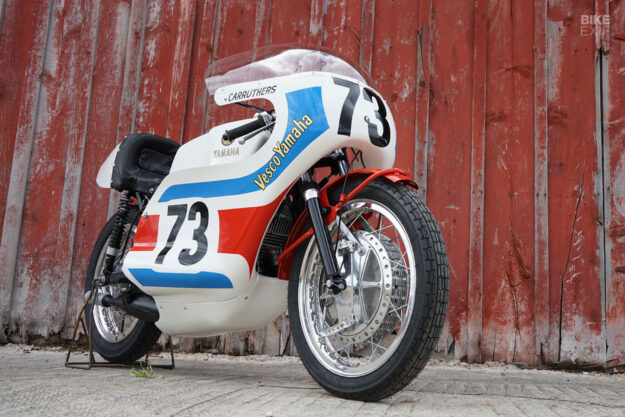This photograph, in landscape mode, captures a Yamaha racing motorcycle positioned against a weathered, faded-red building that resembles a barn, its distressed paint peeling away. The bike, predominantly white with 'Yamaha' in black letters, proudly displays the number 73 on both the front and sides. The name 'Carothers' appears just below the small windshield. The right fairing showcases 'Vesco Yamaha' across a blue accent flanked by a distinctive red stripe, interrupted by the bold black number 73. Notable features include a bright red front fender, a black seat, a black muffler, and chrome disc brakes on its black tires. At the top right corner of the image, the logo 'Bike EXF' is visible in white. The motorcycle stands upright on a white sandy road with the assistance of its kickstand.